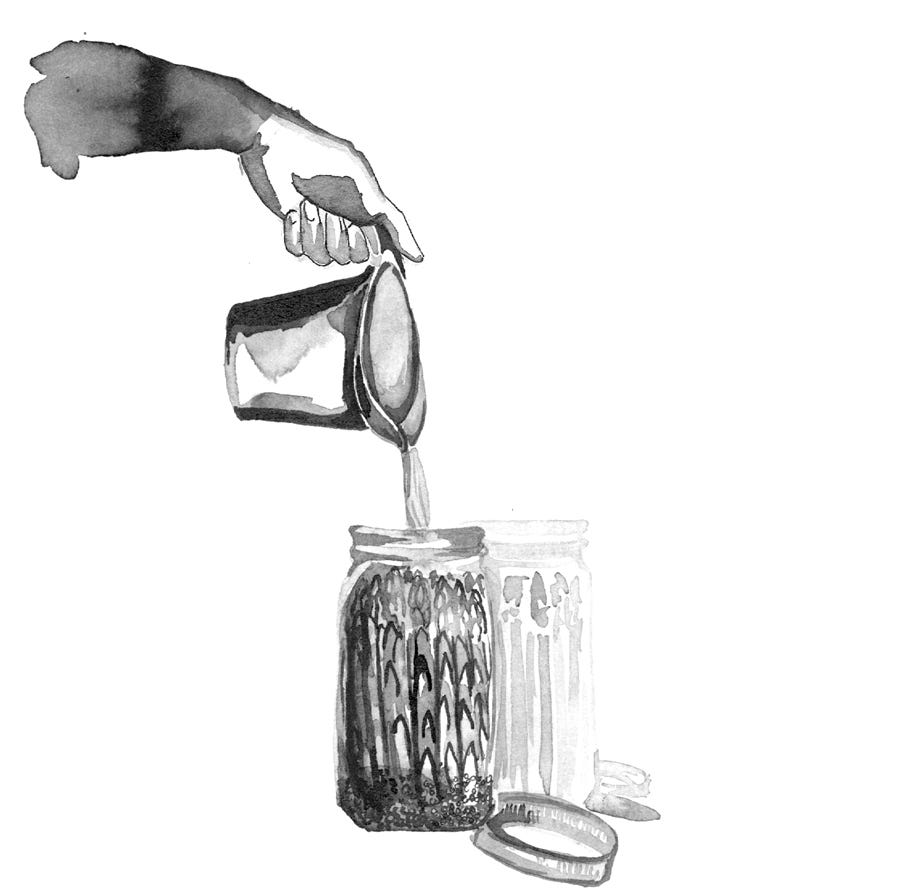The image is a black and white watercolor painting with no background or border, centered on a detailed composition of containers and a pouring action. From the top left, a dark-shaded arm, transitioning to a lighter hand with distinct shading under the thumb, holds a pitcher. The pitcher tilts toward the base of the image, where it pours a stream of liquid into a glass jar. The jar, likely a ball jar, contains what appear to be asparagus stems standing upright, and possibly spices at the bottom. Next to it, slightly behind and to the right, is another jar, shadowy and less defined, giving the impression of an empty or lightly shaded container. Two open jar lids are also present, suggesting they belong to the jars depicted. The entire scene is rendered in shades of black, white, and gray, emphasizing the fluid pouring action and the contrasting textures within the jars.